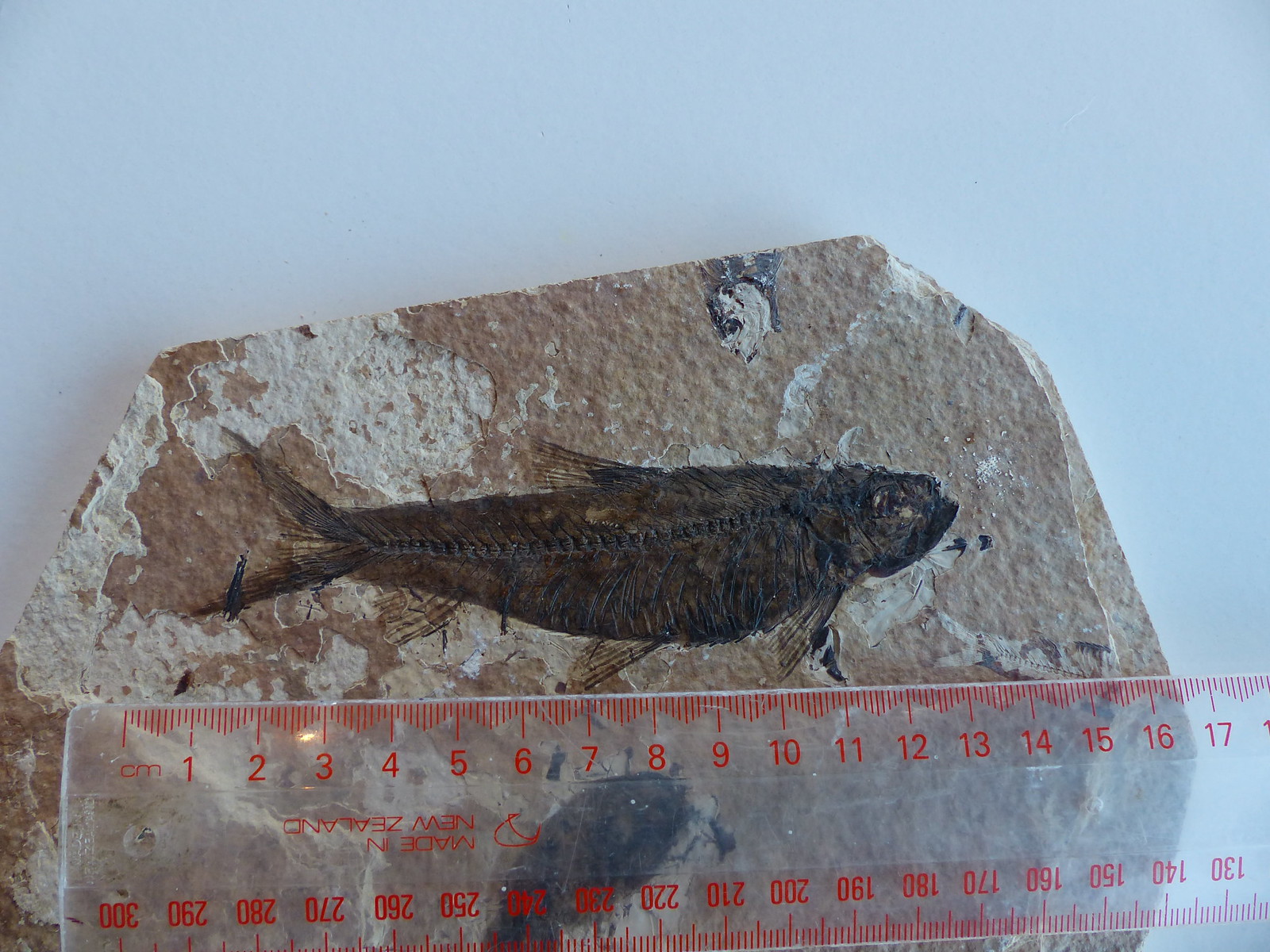The photograph features a fossil of a fish inlaid into a tan and white piece of flat stone, placed on a neutral, white surface. The fossil itself is black and prominently displays the outlines of the fish, including its scales and skeleton. There are also indications of smaller fish fossils, one partially visible towards the top and another obscured at the bottom by a clear acrylic ruler. This ruler, marked with red notches and numbers indicating centimeters and millimeters, measures the main fossil to be approximately 14 centimeters in length. The ruler spans the width of the image from left to right at the bottom, with the fossil positioned centrally on the stone. The only text in the image is on the ruler, which includes measurements from 1 to 17 centimeters along the top and reversed measurements from 130 to 300 millimeters along the bottom, as well as the inscription "Made in New Zealand." The scene appears to depict a scientific measurement process, possibly for a research or educational purpose.